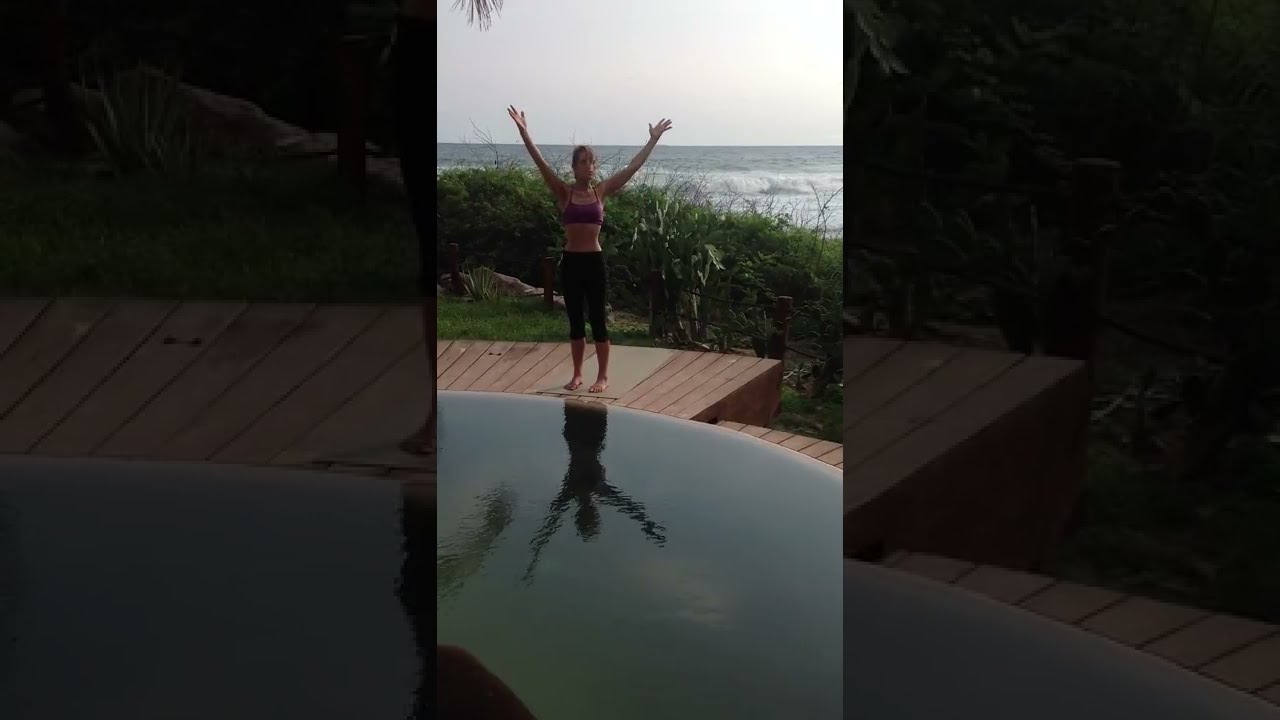This photograph features a slender woman with dark hair standing on a curved, wooden-slatted deck, donning a purple sports bra or bikini top and black capri leggings. She is positioned with her arms raised towards the sky. The image is divided into three vertical panels, with the leftmost and rightmost panels being semi-opaque, magnifying the side sections of the central image. Behind her lies a serene ocean with a backdrop of green foliage and a hill covered in trees. There's a smooth, dark green pool in front of her, which may be part of a trickling fountain or swimming area, where the water appears still and glass-like, reflecting her figure. Rocks and bushes are visible between her and the ocean, contributing to the tropical beach ambiance on this clear yet slightly overcast sunny day. The deck has an orangish-brown hue and seems to carry an Asian influence, suggesting a contemporary design from the last decade.